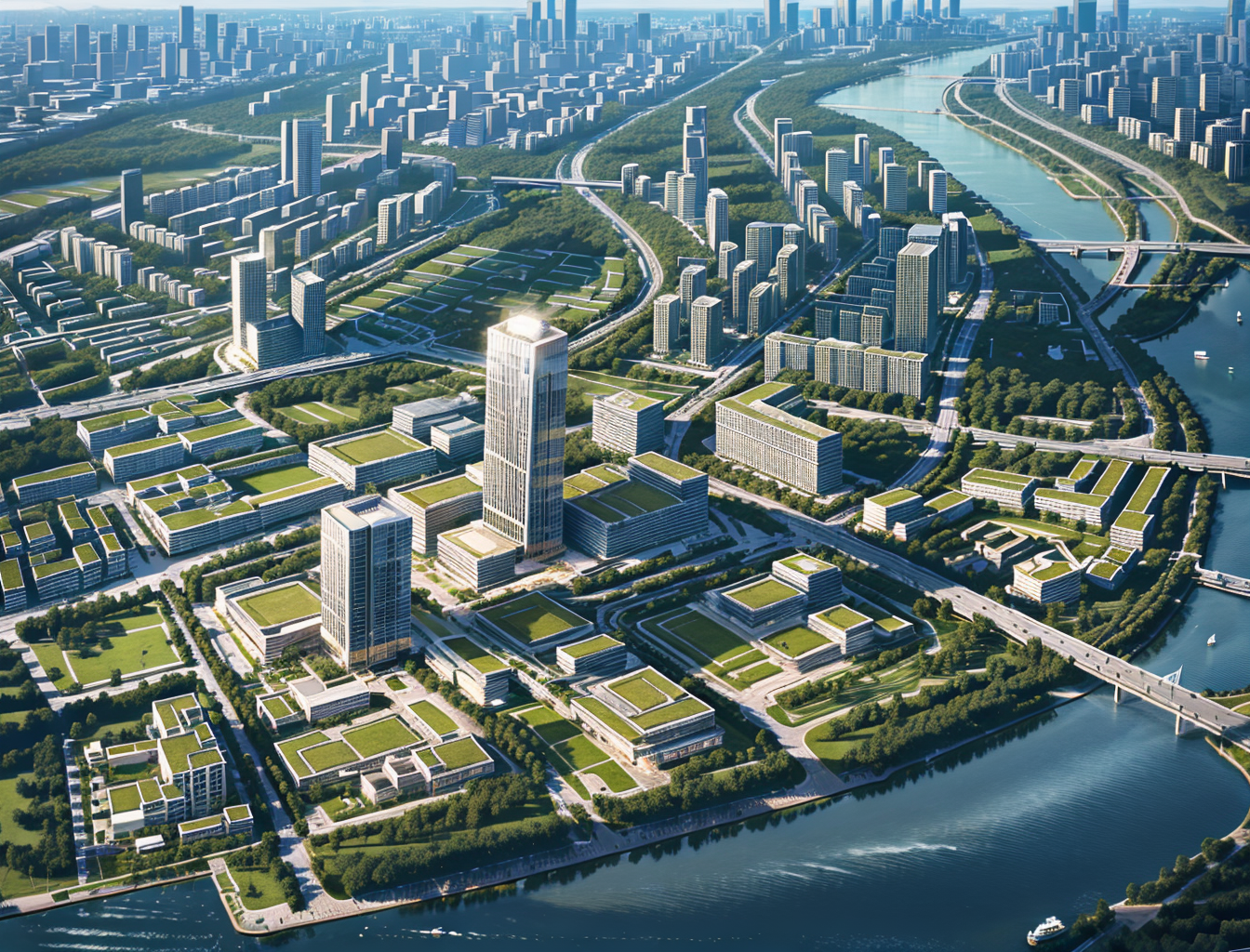This is an aerial artistic rendition of a densely packed city skyline, characterized by its emphasis on green spaces and sustainable design. The city's predominant colors are green, representing grassy areas and trees, and whitish-gray for the buildings, which range from towering high-rises to shorter commercial structures. Each building is intricately detailed, featuring small window areas and verdant roofs covered in lawn, enhancing the city's green aesthetic.

A wide river snakes its way from the upper right to the lower left of the image, with multiple gray road bridges spanning its width, connecting various sections of the city. These bridges facilitate movement across the river, linking the vibrant, densely built-up areas visible in the upper section of the image. The city appears divided into distinct office parks, each comprising numerous skyscrapers and interspersed with highways, streets, and expansive grassy plazas.

The rendering captures a sense of meticulous urban planning, highlighted by the seamless integration of natural elements, implying a utopian vision of an environmentally-friendly urban space. The overall impression is of an animated or 3D-rendered metropolis, with an almost too-perfect, idealized appearance, further suggesting a futuristic or conceptual design aimed at harmonizing urban development with nature.